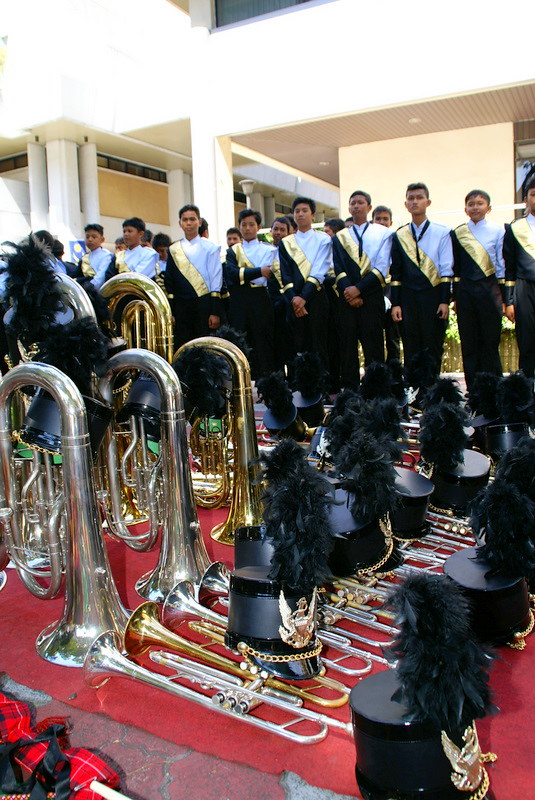The vertically aligned rectangular picture depicts a high school band composed entirely of young men. The boys, approximately 15 in number, have short hair and are dressed uniformly in light blue shirts adorned with diagonal gold sashes, black pants, and standing in orderly rows with their hands either in front of them or at their sides. In the center of the image, lined on a red rug, are various brass instruments, including French horns, tubas, and trombones. Some instruments are lying down, while tubas stand upright. There are also hats with feathers accompanying the instruments on the floor. The background features white pillars and a white wall, suggesting the setting is a conference room or assembly hall. The ground surrounding the rug comprises a red and gray stone pattern. In the lower-left corner of the image, a section of red and black plaid fabric is visible, though its purpose is unclear. The band members face forward, seemingly poised to perform or having just concluded a performance.